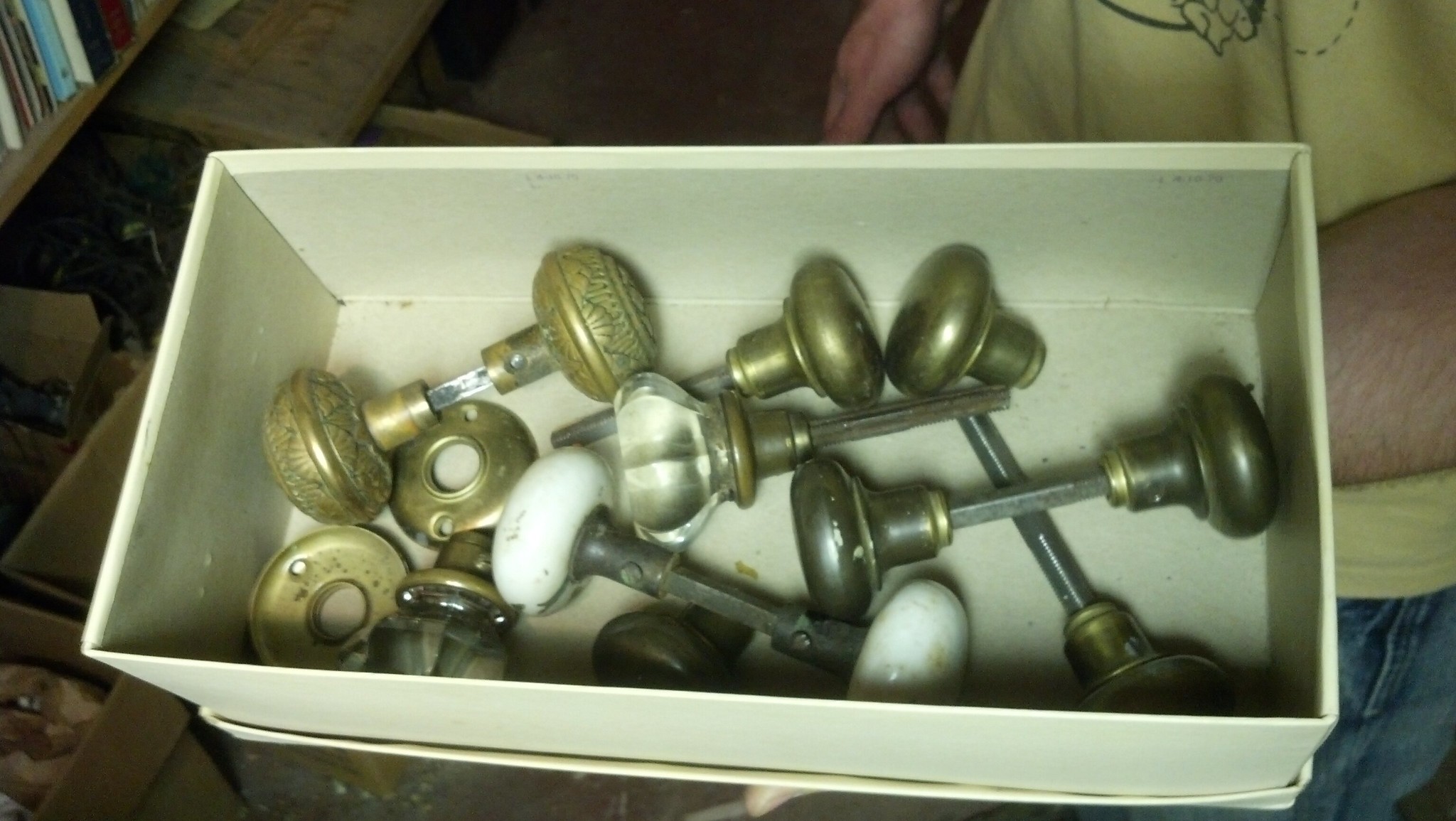The photograph depicts a white shoebox brimming with an assorted collection of antique doorknobs. The shoebox is held by a person's outstretched hand, identifiable by a pink hue, with their arm visible from the right side of the image. This individual is dressed in a yellow t-shirt and blue denim pants, with the fabric of their pocket area just peeking into the frame. In the background, a bookcase with a few books can be seen partially.

Inside the shoebox, a diverse array of doorknobs is neatly arranged. Among them, there is a beautifully ornate brass doorknob with intricate engravings, a pristine porcelain doorknob showcasing two matching white knobs, and a striking crystal doorknob characterized by its transparent facets. Some doorknobs appear to be complete with both knobs attached, while others only display one side. The collection also includes varying colors and materials, such as black enamel and traditional brass, presenting a rich tapestry of design and craftsmanship.